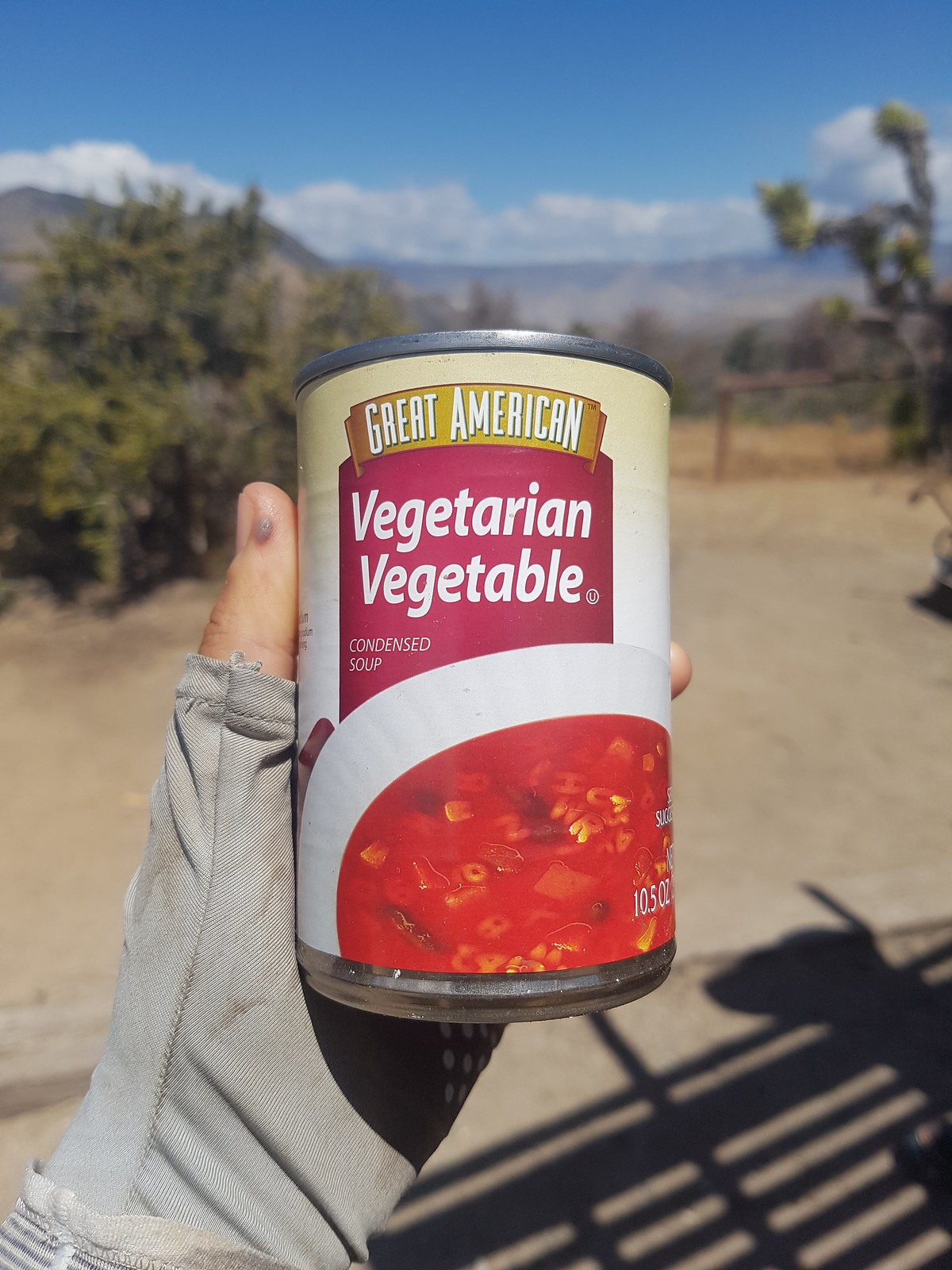In this vertical, outdoor photo, a person with a small, possibly female hand is holding a can of Great American Vegetarian Vegetable Condensed Soup. The hand, adorned with a gray long-sleeved shirt that covers the fingers and thumbs, features a noticeable bruise or blister on the left thumb. The can's label showcases a vibrant bowl of tomato-based vegetable soup, complete with visible noodles and bits of onion, and is designed in purples and greens with a gold banner. The background reveals a blue sky dotted with white clouds, brown gravelly ground, and desert-like flora, including a cactus-style tree on the right and a bush on the left. Shadows cast by a fence and what might be a goat's head add an intriguing element to the scene.